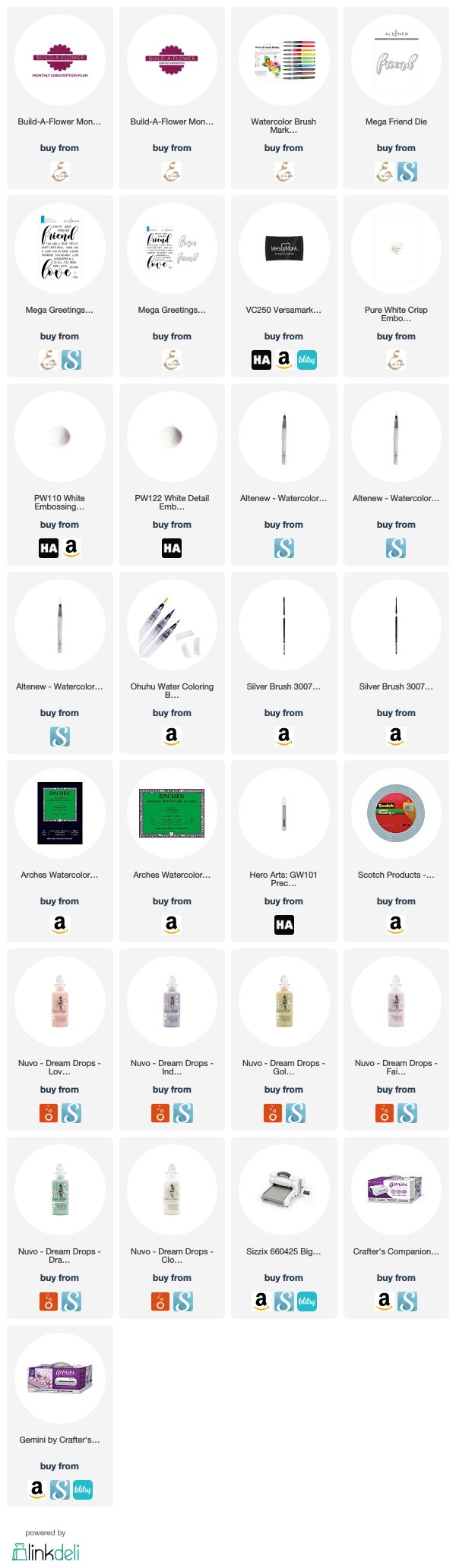This is a screenshot of a product page, displaying a large, organized grid composed of eight rows of items. Each row contains four items, except for the last row, which features only a single item. Each product within the grid is presented with a gray rectangular background. At the top of each rectangle, there is a white circle that showcases an image of the respective product. Below the product image, there is descriptive text providing details about the item. Further down, the text includes a "Buy from" section accompanied by an icon, indicating the retailer from which the product can be purchased. Some of these icons display the recognizable "A" from the Amazon logo, signifying that the item is available on Amazon. This orderly layout provides a comprehensive and visually structured presentation of the products available for purchase.